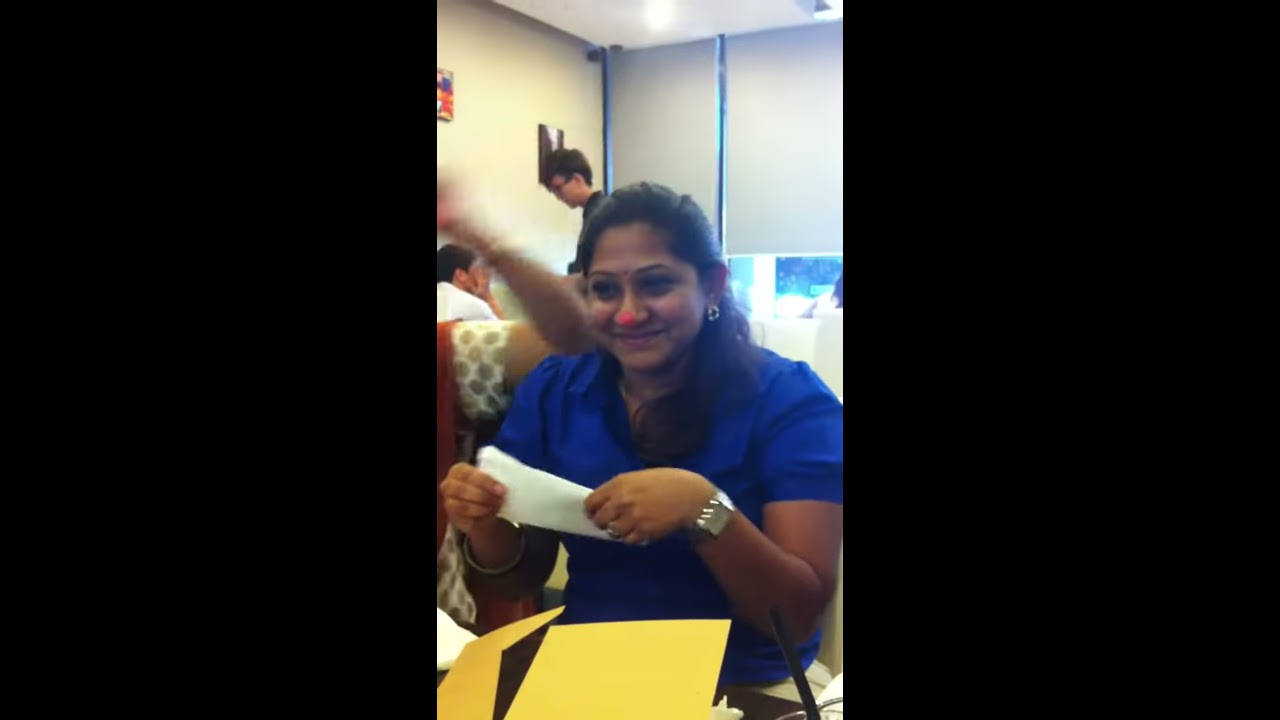In this photograph, we see a young Indian woman, possibly in her thirties, seated at a community center. She is the central figure in the image, wearing a blue blouse, silver and white watch on her left wrist, and a red clown nose. Her brown, straight hair is pulled back, and she has light brown skin. She has a pleasant smile and is looking slightly to the left. In her right hand, she clutches a piece of paper, possibly part of an arts and crafts activity, as there is yellow paper in front of her, and an origami crane can be seen nearby. Surrounding her, other people are engaged in various activities, with glimpses of their arms and conversations visible in the background. The setting is indoors, characterized by a white wall, an open window to the right, and overhead lighting, suggesting it is daytime. The overall scene is lively and communal, capturing a moment of joy and creativity.